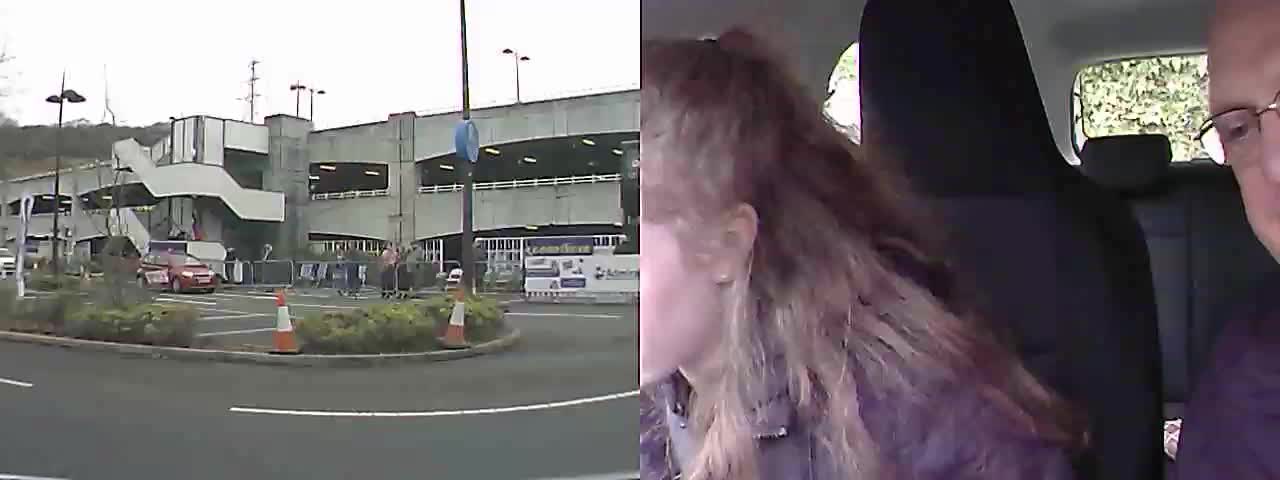The image consists of two separate photographs merged into a single frame. The left photo depicts an outdoor scene, featuring a gray sky and a concrete, two-story parking garage with open spaces. The garage is set against a parking lot that includes an island with bushes and two caution cones. A few cars are visible at the back of the lot. The view appears to be from an entrance lane, emphasizing the parking structure.

The right photo shows the interior of a vehicle, where two individuals are seated in the front. The man on the right, wearing glasses and a purple shirt, is only partially visible from the nose over. He has a fair complexion and appears somewhat heavyset. Seated next to him is a young woman with long, dirty blonde hair, also in a purple shirt, though she is more discernible by her fair complexion, puffy black jacket, and the fact that only her left cheek and part of her body are visible. Both individuals are looking downwards at an unknown object, and the car's upholstery appears to be black vinyl. The overall composition contrasts an exterior urban setting with a personal, interior vehicle scene.